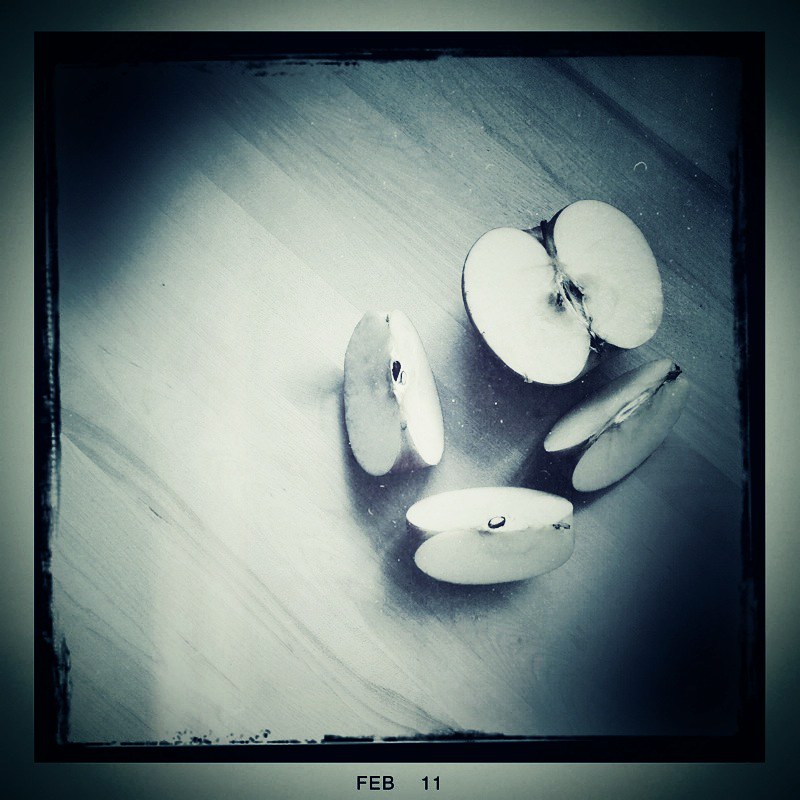The image is a black and white, square-shaped photograph with a black border, resembling a vintage Polaroid style. It captures a sliced apple arranged artfully on a wooden surface. The apple has been cut in half, with one half further divided into three sections, all positioned with the cut sides facing the camera, revealing the seeds and core. The edges of the photo are darkened by shadows, especially in the upper left and lower right corners. The center of the image is illuminated, likely by a flash. At the bottom of the photograph, the date "Feb 11" is prominently displayed, adding a timestamp to this artistic composition. The entire scene is in grayscale, emphasizing the textures and contrasts between the apple, wood grain, and shadows.